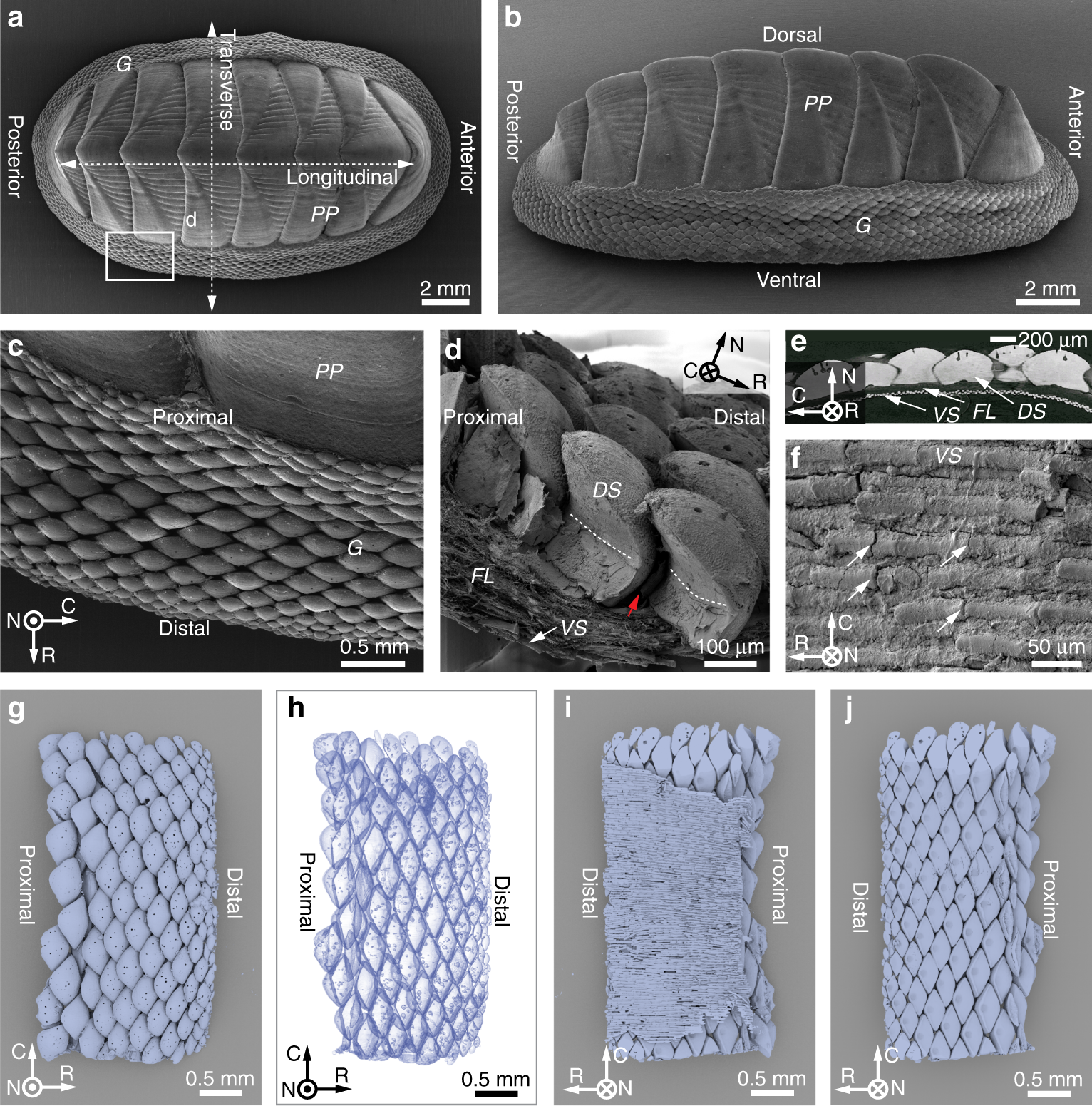This image collection, possibly from a scientific publication, contains ten microscopic photographs arranged in three rows. The top row features images labeled A and B, the middle row includes images C, D, E, and F, and the bottom row comprises images G, H, I, and J. Each image captures different perspectives and parts of an unidentified specimen, possibly fish or snake scales, with various labels indicating orientations and sections.

In the top row, image A, which looks like the top of a bug, is annotated with "anterior," "posterior," "transverse," and "longitudinal." Image B, showing a side view, is labeled "dorsal," "anterior," "ventral," and "posterior." Images C and D are marked with "proximal" and "distal," with C resembling a scale. E and F are smaller squares without detailed identification.

The bottom row images, G, H, I, and J, are pale blue. Images G and H have proximal on the left and distal on the right, with G's background being gray and H's background white. Images I and J, also gray, are labeled with distal on the left and proximal on the right. This meticulous array of images showcases various shapes and orientations, providing an extensive view of the specimen's morphological diversity.